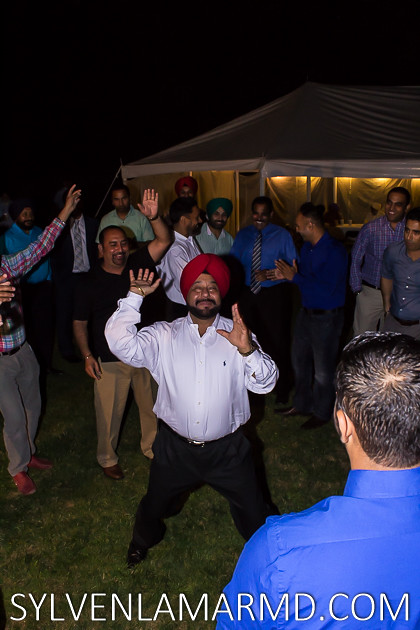The photograph, sourced from sylvanlamardmd.com, captures a vibrant nighttime outdoor celebration with a pitch-black sky overhead. The scene is set in a flat grassy field, where a large group of men, most of Indian descent and some in suits, enjoy the festive atmosphere. Central to the image is a jubilant Indian Sikh man, easily identifiable by his red turban, white button-up shirt, and black pants, exuberantly dancing with his hands raised. His joyful energy is mirrored by the surrounding crowd, where several men cheer him on, some clapping and others smiling broadly.

Behind the revelers stands a well-lit pavilion tent, its white poles and strings securing the structure. The tent, with some of its walls rolled up, reveals a table inside and emits a warm yellowish light, contrasting with the green-colored roof. Within the crowd, various men are visible, dressed in a mix of shirts, with a few also donning turbans. One individual stands with his back to the camera, adding depth to the composition. Overall, the image beautifully encapsulates a moment of shared joy and cultural celebration under the night sky.